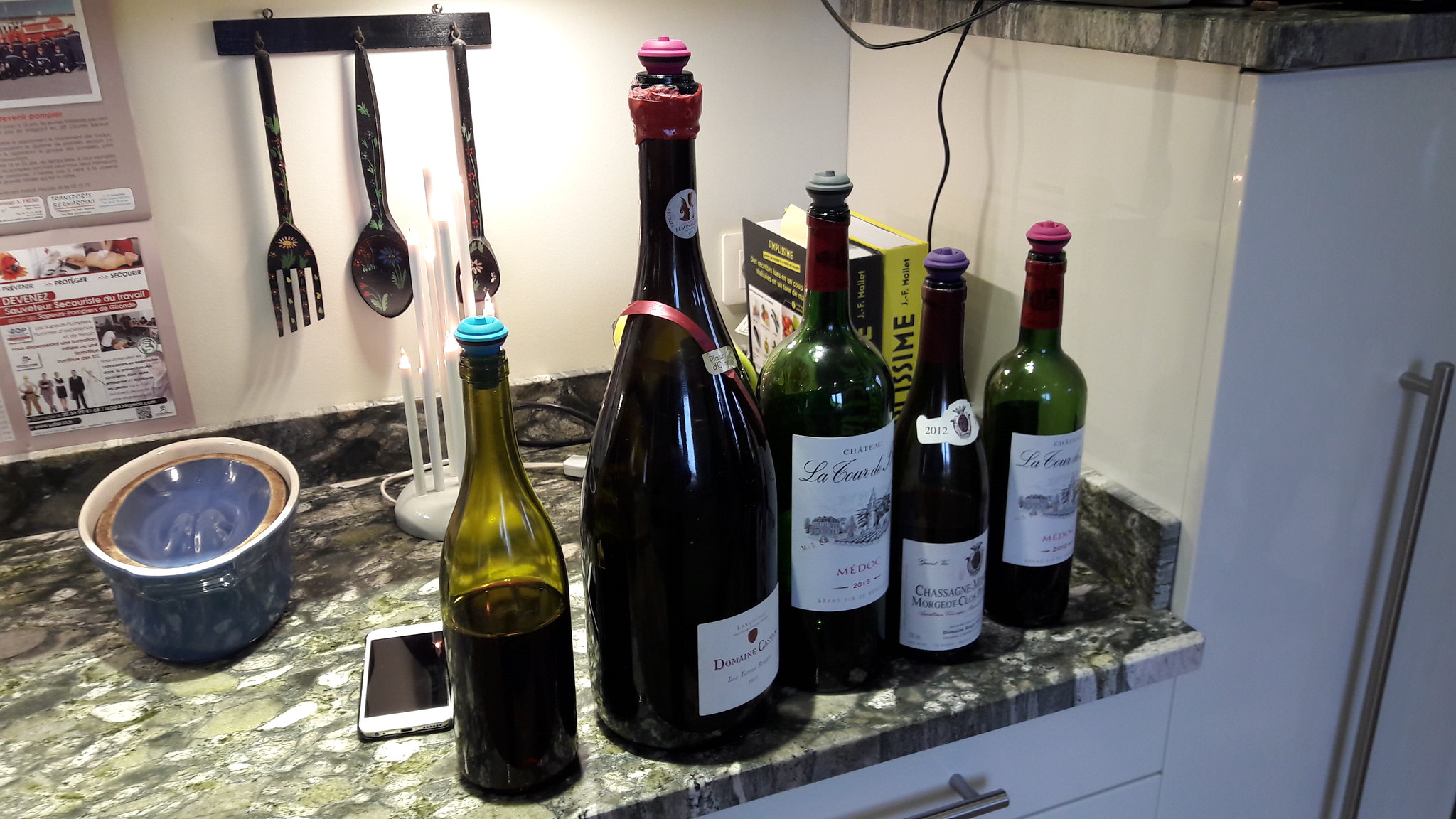The photograph captures a detailed view of a kitchen setup with a grey and white marble countertop as the focal point. On the countertop, there are five wine bottles, each topped with a unique, colorful reusable stopper in light blue, pink, gray, purple, and mauve. The leftmost bottle, which is green and either half-empty or half-full depending on your perspective, is unmarked. Adjacent to it is a white smartphone, likely an iPhone. The second bottle is a large, black bottle with a white label and a distinctive red ribbon attached. Next to it stands a dark green bottle with a white label, a black bottle with white labels, and another green bottle, all adorned with white labels. Positioned behind the bottles, there's a ceramic pot with handles and an inverted lid. The background features a white wall adorned with plastic utensils, including a combination fork and ladle, a spoon, and a slotted spoon, as well as some posters or signs. To the right of the countertop is a white fridge and matching cabinets and drawers, completing the kitchen scene.